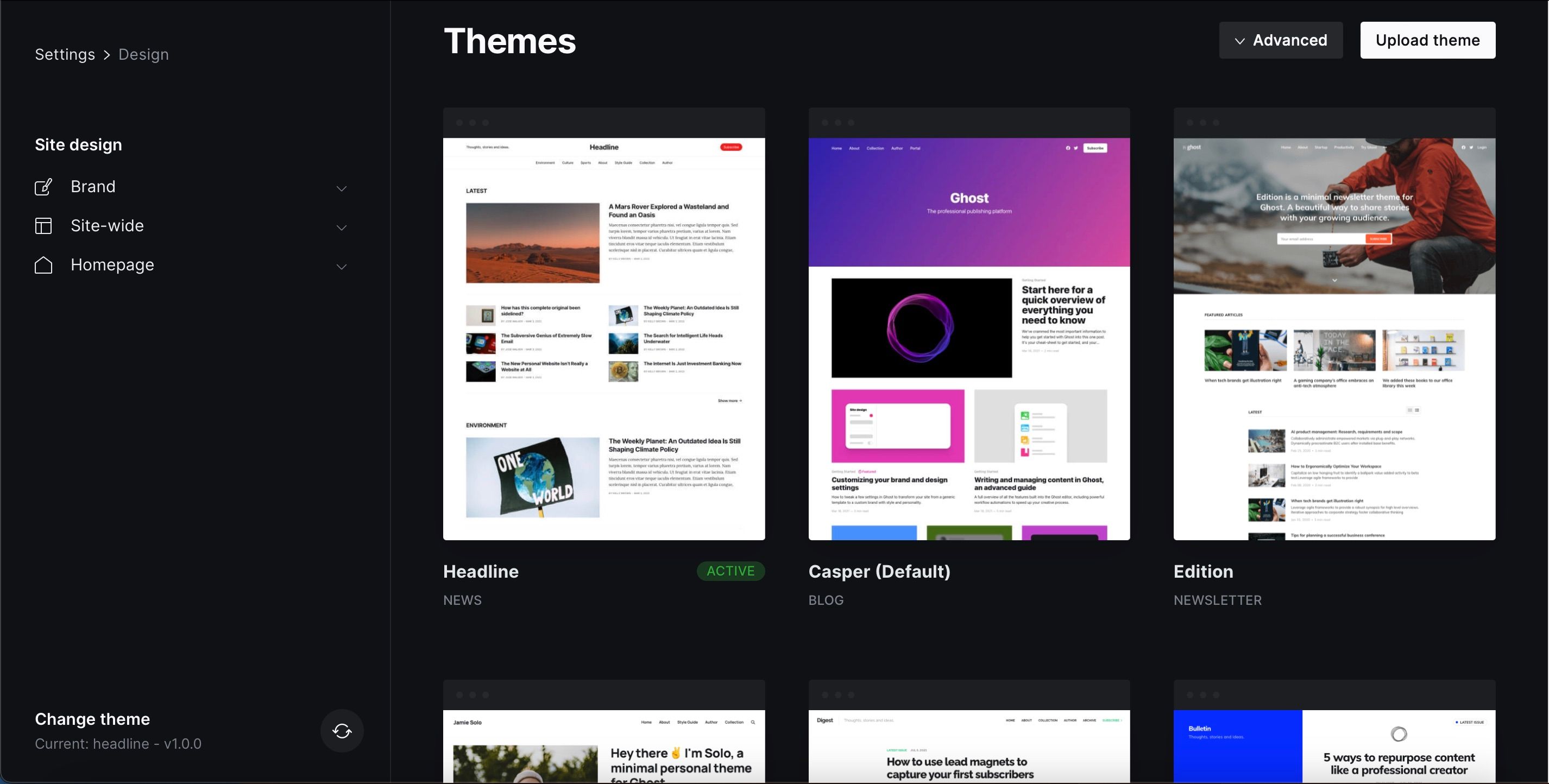Screenshot Caption: A Comprehensive Website Development Interface

The image is a screenshot of a website development platform designed for users who seek to publish or develop their own websites effortlessly, without requiring extensive web development knowledge. The platform offers a plethora of themes and templates for easy customization. 

The background of the interface is a dark gray or black, giving it a sleek, modern appearance. On the left side of the screen, a vertical menu lists options for site design, including sections labeled "Brand," "Site-wide," and "Home Page," allowing users to navigate different areas of their website. 

In the bottom-left corner, the words "Change Theme" are displayed in white text, with "Current: headline-v1.0.0" appearing below in gray text, indicating the currently selected theme.

Across the center and right sections, the available themes are displayed prominently. At the top center, the word "Themes" is presented in large white text. Below this heading, various theme options such as "Headline," "Casper (default)," and "Edition" are showcased with corresponding screenshots. These images provide a preview of what each theme would look like when applied to a user's website, facilitating informed selection.

In the top-right corner of the interface, two additional options are available. A gray box with white text labeled "Advanced" is situated next to a white box with gray text labeled "Upload Theme," enabling users to either choose new themes from an advanced selection or upload custom themes of their own.

This comprehensive interface ensures that even those with minimal web development skills can create professional-looking websites effortlessly, tailored to their personal or small business needs.